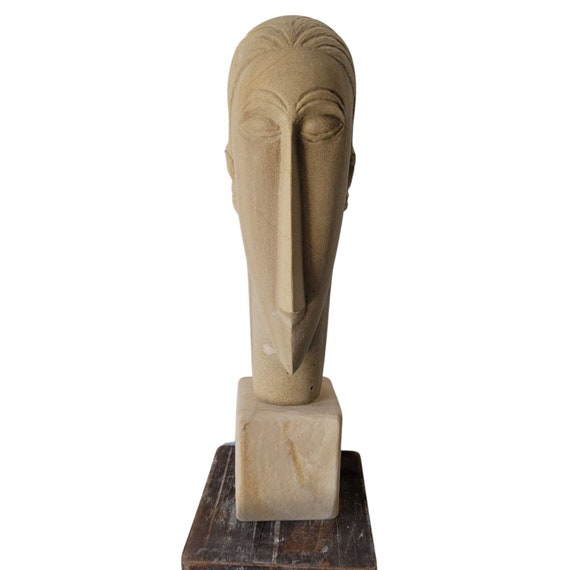This sculpture, likely crafted from a matte gray-beige stone, depicts a highly stylized and elongated human head. The head is disproportionately long and narrow, with notably exaggerated features. The nose is unusually extended and angular, nearly a foot in length, seamlessly leading to a sharply pointed chin that enhances the sculpture's oblong appearance. Despite possessing facial features like eyes, arched eyebrows, and simple etched lines representing hair, the piece forsakes realistic anatomical accuracy for a more abstract form. The eyes appear closed, contributing to the stylized aesthetic. The head is mounted on a square pedestal, possibly marble or wood, which rests on a larger, darker base, providing a visually contrasting platform for the statue. The total height of the sculpture, including its pedestal, is estimated to be two to three feet, reinforcing its imposing presence.